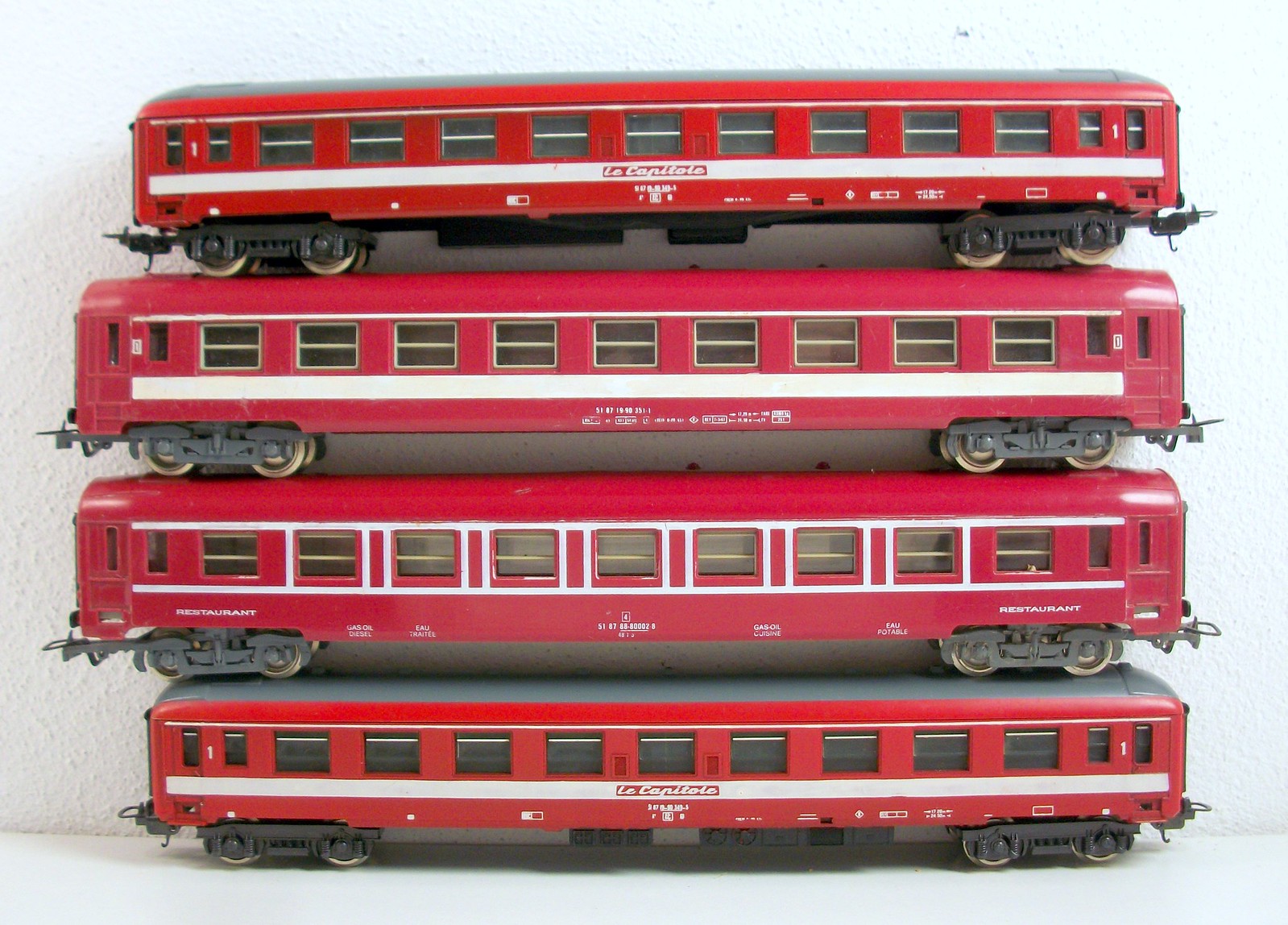The image presents a collection of four model train coaches, meticulously stacked on a white floor against a concrete wall, also painted white. Despite the absence of the train's front part, each coach displays a distinct design while maintaining a unified red theme. The bottom coach features a broad white rectangle beneath darkened windows, with red text on a white background, potentially spelling "La Conitole." It is distinguished by its silver or gray roof. The second coach, similar to the first, but with a red rectangle resembling a ladder between the windows, exhibits subtle design variations. The third and fourth coaches closely mirror the first, sporting a prominent white rectangle beneath the windows accompanied by a smaller one above. Interiors, albeit slightly visible, hint at beige shading, possibly from blinds or lighting differences, emphasizing their model toy nature through their plastic texture and sheen.